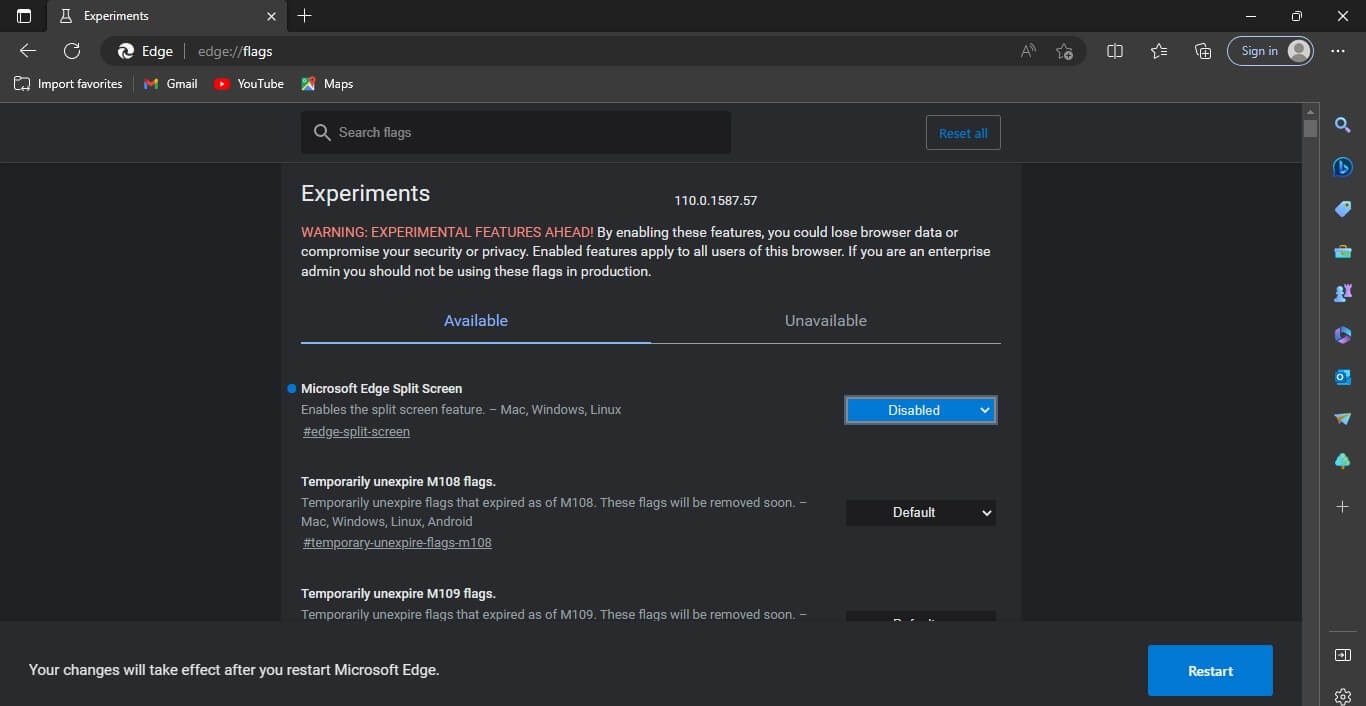This is a detailed description of a visual interface from a user's homepage, characterized by its dark, nearly black color scheme. 

At the top, there's a prominent black border. The far left corner includes a small black square. Next to it, a gray section extends about an inch and a half to the right, followed by a continuation of the black border. In the top left corner within the black section, a white-outlined box is visible. Adjacent to this box in the gray section, the word "Experiments" is displayed. Further to the right, outside the gray segment and back in the black border, a white plus sign can be seen. The right end of the top border is adorned with a series of white icons: a white 'X', a white square, and a white dash.

Beneath this top border on the left side, there are two white icons; a left-pointing arrow and the refresh button. The search bar, displaying "edge://flags", is situated centrally. On the right of the search bar, the interface features a 'sign-in' tab, a 'star' tab, and a 'favorites' tab below it.

Further down on the left side, a small square labeled "import favorites" is visible, followed by an icon 'M' representing Gmail, a YouTube icon labeled YouTube, and a Maps icon labeled Maps. Below this section, roughly two inches from the left, there's a black search space. Around two inches to the right of this is another black tab with "Reset All" written in blue.

Running down the side are approximately 12 different clickable tabs, each leading to various sites. Under the search bar, the word "Experiments" is prominently displayed, with a follow-up warning, "Experimental Features Ahead," spanning three lines. Below this warning, in blue text, the words "Available" appear on the left side, while "Unavailable" is noted in gray on the right side. Three tabs are aligned underneath: the first one reads "Turned On."

This comprehensive layout forms a part of the interface, providing a structured navigational experience.